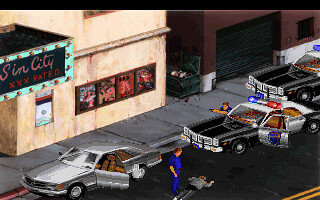The image depicts a retro-style scene reminiscent of video games from the 1980s or early 1990s. Dominating the scene is the exterior of a store featuring a neon sign that reads "Sin City" with "XXX rated" below it. The store's facade is constructed from a weathered, yellowish stone, further adorned with multiple posters, likely advertising various movies or events.

In the immediate foreground, a sidewalk extends alongside the store. An alleyway in the background reveals a gritty urban landscape with a dumpster and a red building characterized by a warehouse-style door. The intense scene unfolds with a police car parked outside the store, with a police officer aiming a gun. Nearby, a gray car has its doors flung open, suggesting a hurried exit or confrontation. A figure dressed in blue stands over another figure in gray, who lies motionless on the ground. Another police car is visible behind the first, indicating a significant law enforcement presence.